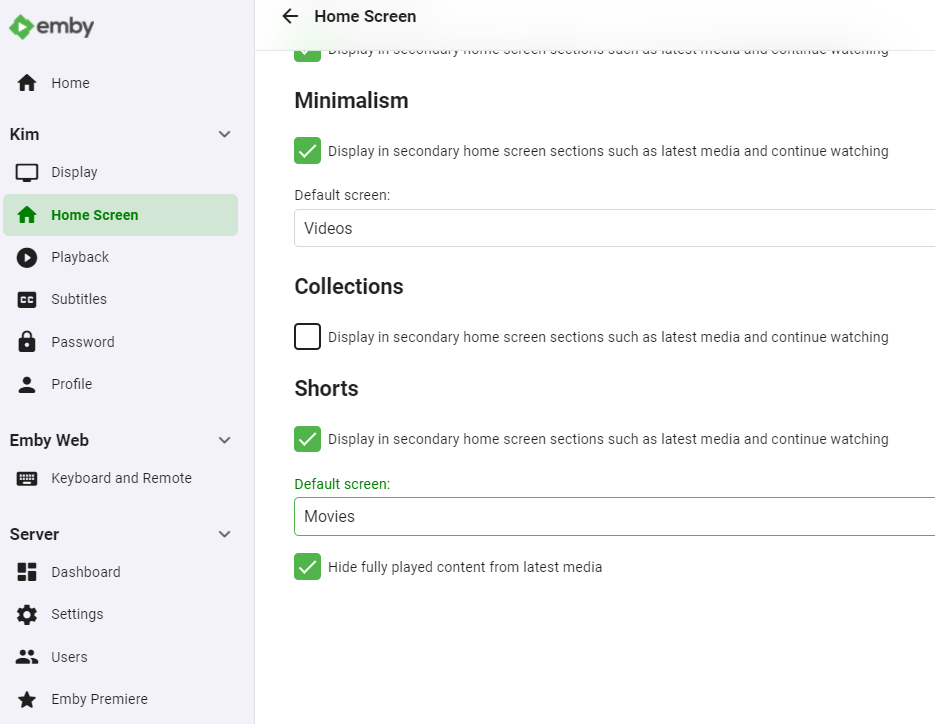The image appears to be a screenshot of a section of a website, specifically the navigation and settings panel of an application. On the left-hand side, there is a light grey column featuring a vertical menu. At the top of this column is a green diamond-shaped icon with "NB" written in black. Below the icon, the menu includes various options, paired with small black icons, including: 

- Home (with a black house icon)
- Kim (with a downward arrow)
- Display (with a display icon)
- Home Screen (highlighted in green)
- Playback
- Subtitles
- Password
- Profile
- NB Web
- Keyboard and Remote
- Server
- Dashboard
- Settings
- Users
- NB Premiere

On the right-hand side of the screenshot, the top section reads "Home Screen" in black and white, accompanied by a back arrow. Below that, partially obscured text is visible, suggesting an interface hidden under the panel. Only the edge of a square checkbox is discernible, with the bottom of the text unreadable. 

Under this section, the word "Minimalism" is displayed prominently, followed by a green ticked checkbox. The accompanying text reads, "Display in secondary home screen sections such as Latest Media and Continue Watching."

Further down, under "Default screen," there are several options each associated with tick boxes:
- "Videos," followed by a toggle that is not ticked, with the same text about displaying in secondary home screen sections.
- "Collections," with an unticked checkbox.
- "Shorts," with a ticked checkbox displaying the same secondary home screen information.

Finally, the topic "Movies" is presented with a partially visible green-outlined rectangle and a ticked green checkbox beneath it. The text here states, "Hide Fully Played Content from Latest Media."